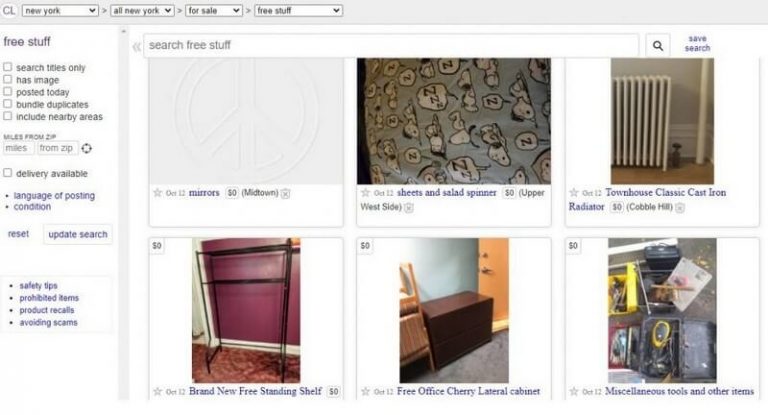The image showcases a website dedicated to listings of items for sale. Prominently on the left side of the image is a navigational menu designed to aid users in refining their searches. At the top of the menu, the "Free Stuff" category is selected, providing options to search for items by specific criteria. The search filters include "image posted today," "bundle duplicates," and the option to "include nearby areas." Users can also specify the search radius in miles from their zip code, check a box for "delivery available," choose the "language of the posting," and filter by "condition." Beneath these filters, buttons labeled "reset" and "update search" allow users to refresh their search criteria. Additionally, the menu offers safety tips, lists prohibited items, and suggests ways to avoid scams.

To the right of the menu, the image displays six item thumbnails arranged in a 2x3 grid. In the top row, the first thumbnail features "mirrors" with a visible outline of a peace symbol. Next, the second thumbnail displays "sheets in a salad spinner," where the sheets are gray and adorned with Snoopy. The third thumbnail showcases a classic cast iron radiator heater. In the bottom row, the first thumbnail highlights a "tall standing shelf," followed by a "cabinet," and finally, a set of "tools." Each item is accompanied by clear images, helping users to see what is available at a glance.